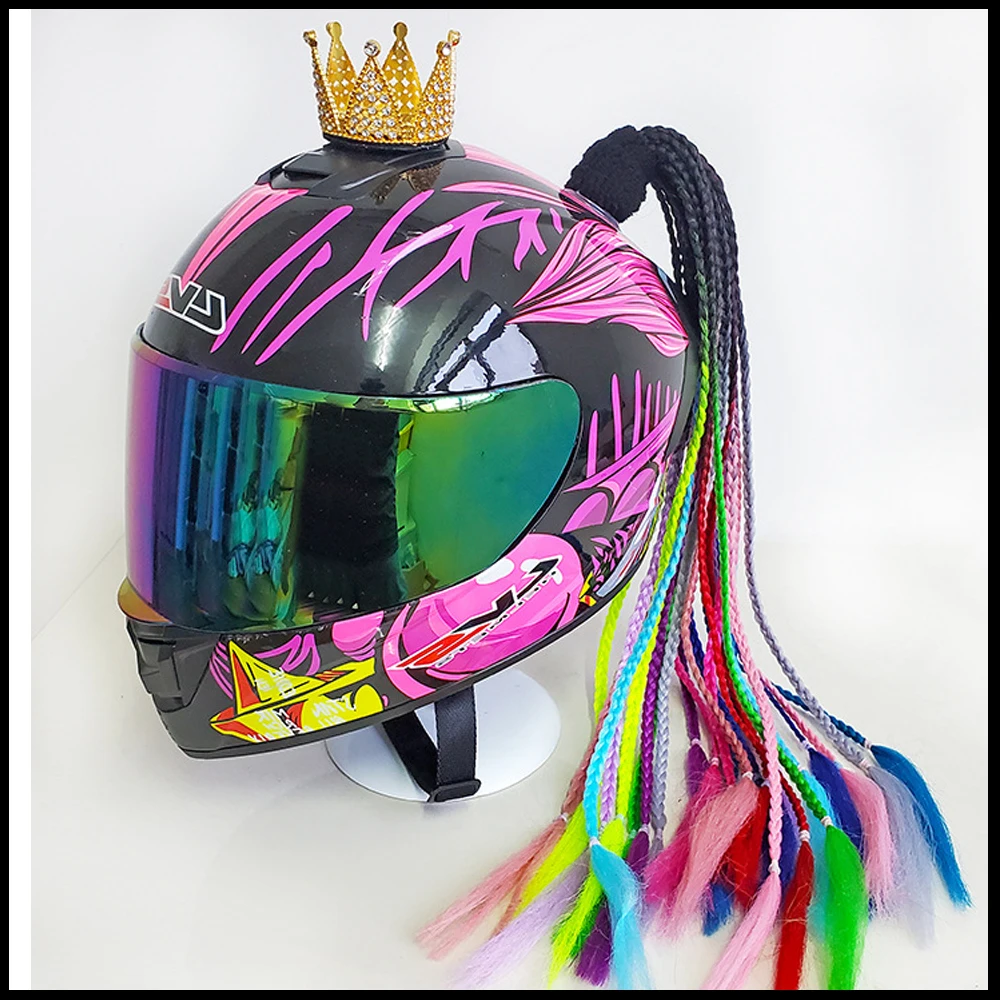This professionally displayed image features a striking motorcycle helmet with a predominantly black design adorned with elaborate pink and yellow patterns. The helmet, positioned slightly to the left against a pristine white background, boasts a crown at its pinnacle—a small gold accessory studded with delicate white diamonds. Adding to its unique flair, the helmet has multiple braided ponytails cascading from the back. These braids start as black at the top and transition into a vibrant array of colors, including fluorescent yellow, bright green, light and dark blue, hot pink, purple, red, and gray. The face mask is rainbow-colored, adding to the helmet's festive and eye-catching aesthetic. A black chin strap secures the helmet, completing its intricate and colorful presentation.